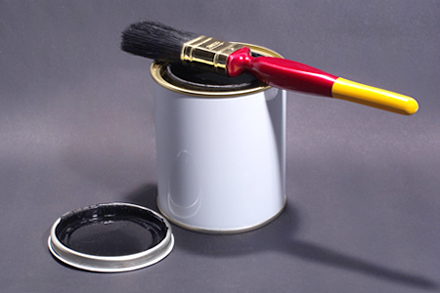In this color photograph, set in a landscape orientation, a pristine white, unlabeled cylindrical paint can takes center stage against a light gray backdrop. The can, accented with golden trim on both the top and bottom, has its lid removed and placed upside down to the left; the interior of the lid is coated with black paint, suggesting the contents are a dark, glossy shade. Resting diagonally across the open can is a paintbrush, featuring a distinctive handle with a shiny yellow base transitioning to a cherry apple red upper half. The paintbrush's bristles, which are oriented towards the top left corner, are highlighted by a shiny gold ferrule. A subtle shadow extends from the can and the handle of the brush, cast towards the lower right of the image, adding to the realism and depth of the composition.